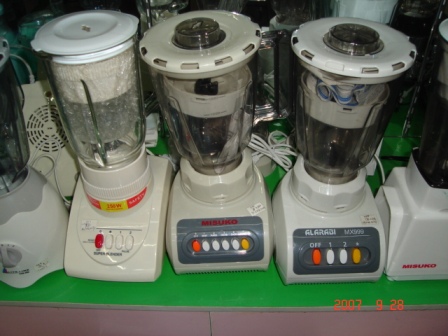This photograph captures five distinct vintage blenders arranged side-by-side, showcasing their retro design elements. Each blender boasts a large, boxy base adorned with multicolored buttons that evoke a 1970s aesthetic, paired with a glass pitcher placed on top. The blenders, although not identical, share a common cream-colored base and white lids, contributing to a cohesive yet varied collection. The scene is set on a green foam mat atop a gray shelf or table, which may hint at a thrift shop or garage sale setting. The image, which seems to be from a security camera, also includes a timestamp at the bottom right reading "2007-09-28," adding a layer of historical context to the visual.